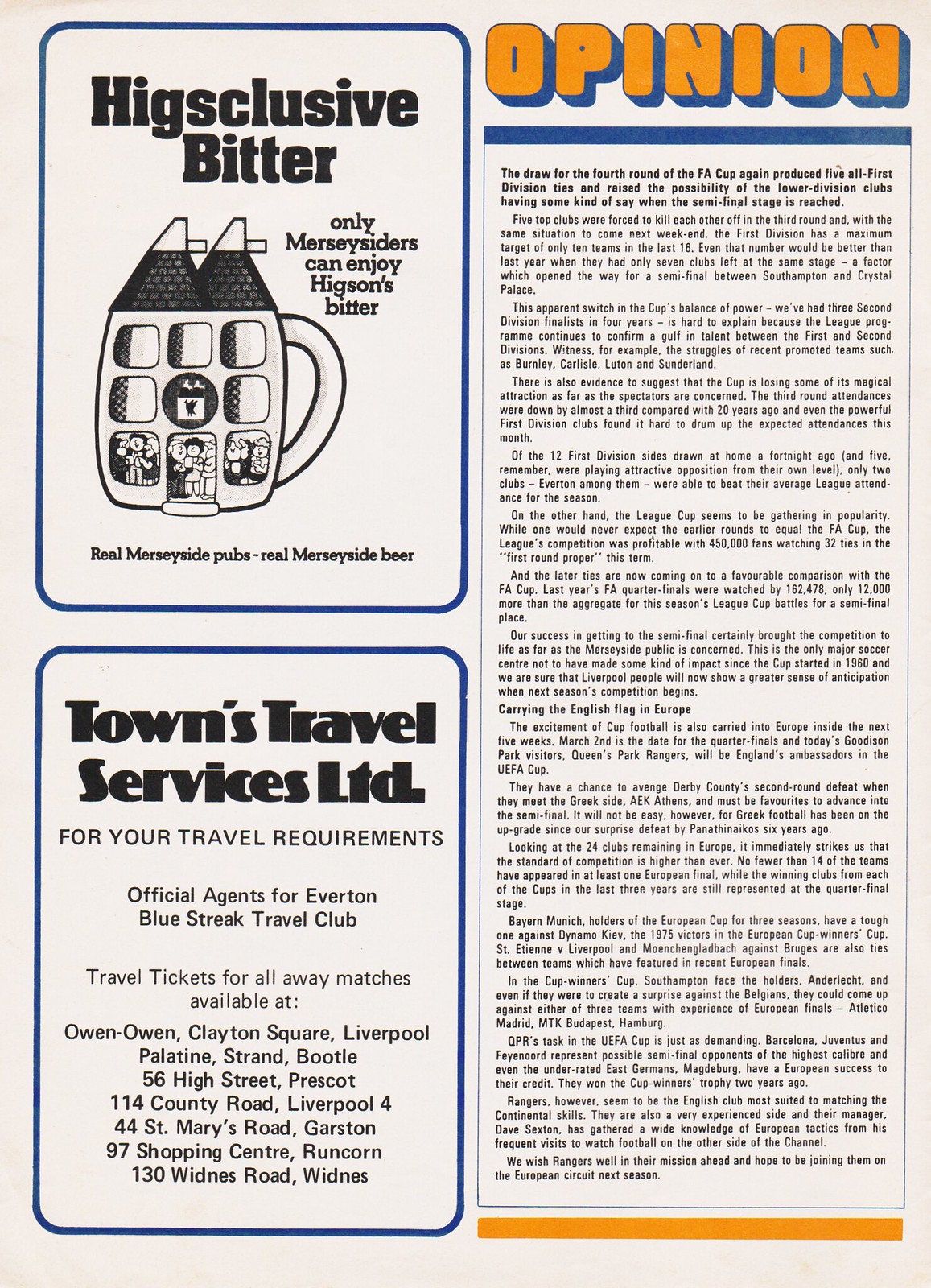The image is a detailed page from a magazine. The background is primarily white with a cream hue, and the content is divided into three distinct sections. On the left side, there are two blue-bordered white rectangles that house advertisements. 

The top advertisement promotes "Higgsclusive Bitter" with the slogan "Only Merry Ciders Can Enjoy Higgson's Bitter" in black text. Below the text, there is a whimsical cartoon depiction of a beer mug designed to look like a house. The mug features eight windows at its base, a central doorway with cartoon figures peeking out, and two black, triangular roofs at the top. The ad concludes with the words "Real Maryside Pubs, Real Maryside Beer" in black text.

The bottom advertisement is for "Towns Travel Services, LTD." It features bold black text on a white background inside a blue border. The message reads "For Your Travel Requirements, Official Agents for Everton Blue Street Travel Club" followed by details about travel tickets for away matches and the addresses of various locations such as Owen Owen, Clayton Square, Liverpool, and others.

On the right side of the page is a detailed article. At the top right corner, in orange font with a blue border, the word "Opinion" is prominently displayed. Below this is a blue-bordered white rectangle containing several lines of black text describing the draw for the fourth round of the FA Cup. The article suggests that lower division clubs may have an impact when the semi-final stage is reached, with first-division teams potentially reduced to a maximum of ten in the last sixteen. The text continues beyond the visible portion, indicated by the phrase "and then it reads on."

The article is composed of approximately five to six paragraphs of small black text, suggesting a comprehensive analysis. The page layout is neatly organized, with a horizontal orange strip at the bottom right corner, providing a balanced finish to the page design.

Overall, the combined captions highlight the clear division between the advertising content on the left and the detailed opinion piece on the right, with distinctive and colorful design elements that make each section stand out.